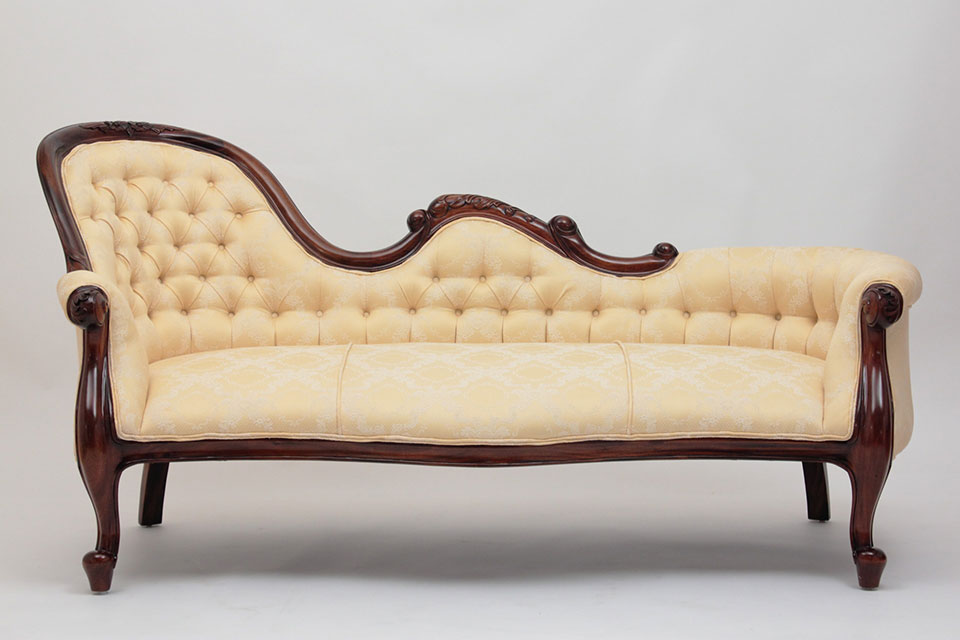This image features a vintage chaise lounge, centrally placed against a completely white or grayish-white background. The chaise lounge boasts a rich dark wood frame, likely cherry, with ornate carvings, possibly floral, running along its length. The upholstery is a cream or beige colored fabric, meticulously maintained and featuring a woven design with tufted buttons that create a quilted effect.

The lounge design is distinctly antique, reminiscent of the 1800s or possibly the French colonial period. The left side of the chaise lounge includes a tall backrest, beautifully curved and adorned with a small hump in the middle, while the middle section has a lower armrest. The right side slopes gently down to where the feet would rest. This creates an elegant flow with wavy curves that add a sophisticated touch to its overall appearance.

The wooden legs of the chaise lounge are meticulously crafted, with the two front legs being bent and ending in small knobs, while the back legs remain straight. This striking piece marries intricate design with refined comfort, capturing the essence of timeless elegance.